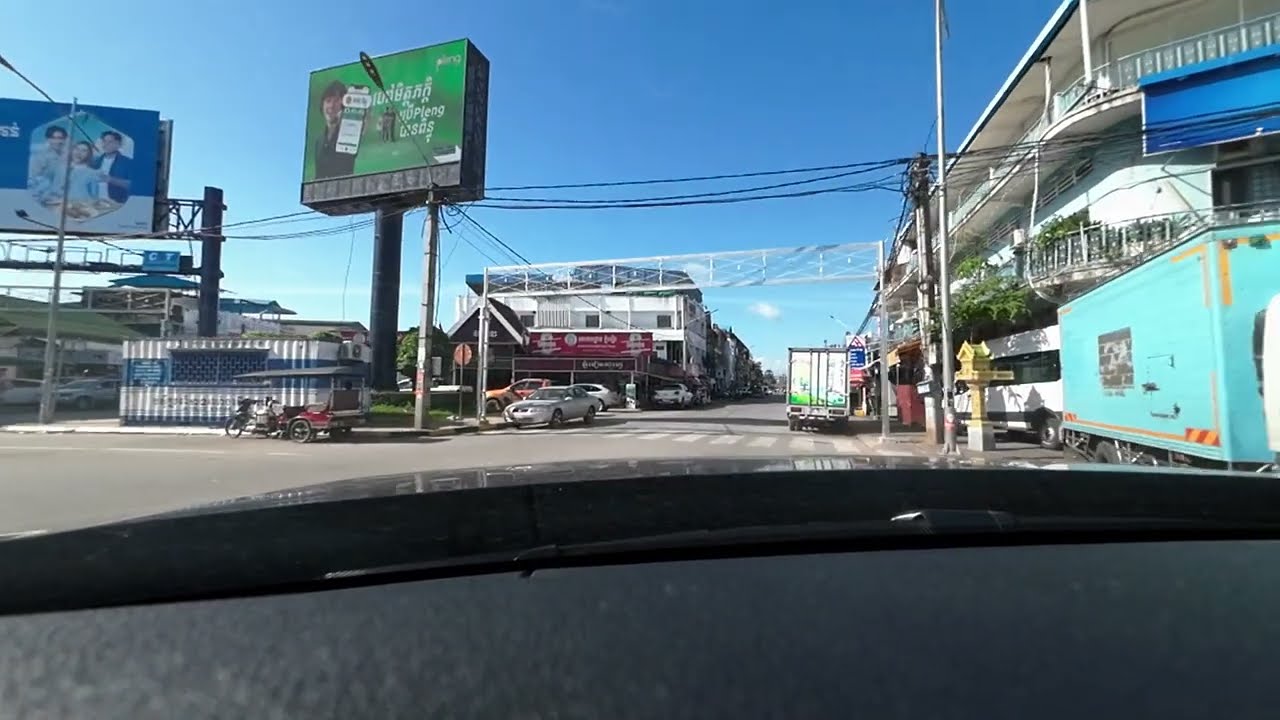The photograph, taken from the dash cam of a vehicle heading straight through a bustling urban intersection, captures a vivid cityscape, likely somewhere in Southeast Asia. The scene is dense with activity and details. At least a four-way intersection stretches out ahead, with multiple vehicles including box trucks, cars, bicycles, and even a motorbike navigating the streets. Two prominent billboards dominate the view; one with a green background and white lettering features a man holding a phone, while another blue billboard showcases a photo of three people. 

Near these advertisements, a small blue and white trailer sits adjacent to a cart. A white and green truck is parked across the street, while to the right side, another blue truck is stationed outside a building. This building features several stories, adorned with a balcony that has a white railing, a blue overhang, and some plant decorations. Light poles and electrical wires crisscross above, typical of a lively city atmosphere, and trees are dotted along the sidewalks. The intersection is also marked with a well-defined crosswalk, and a fire hydrant is visible, adding to the intricate urban setting. The presence of Asian characters on signage suggests this vibrant street scene is situated in a Southeast Asian city, enhancing the cultural context of the image.